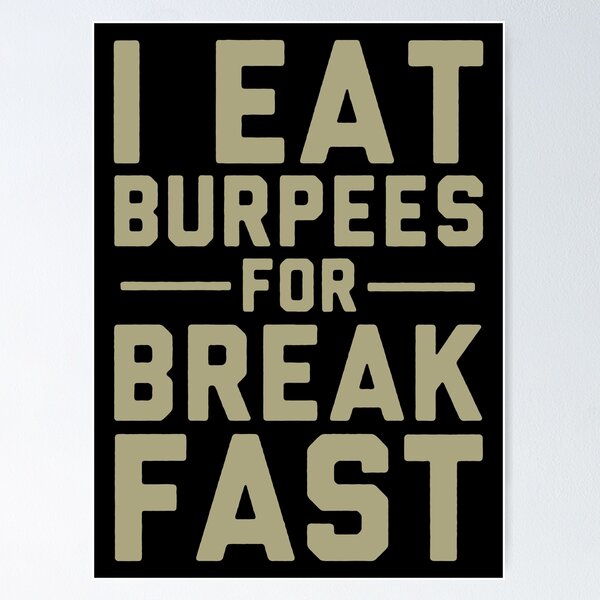The image depicts a wall-mounted sign with a sleek, modern design. The background of the sign is entirely black, providing a sharp contrast to the bold, gold-tan text that spans the sign from top to bottom. The text, starting from the upper left corner, reads in a stylized sequence: "I eat" at the top, followed by "burpees" on the next line, then a dashed line, then "for," another dashed line, and finally "breakfast," split into "break" and "fast" on two lines. This arrangement gives the message a rhythmic, dynamic feel. Surrounding the central text is a thin, white border that delicately frames the artwork. The colors featured are blacks, grays, whites, and a dull gold, creating a sophisticated and somewhat industrial look. The overall setting suggests that this sign is intended as a motivational piece, perfect for hanging on a wall in a gym or fitness space.